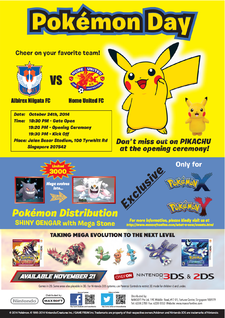The image has a vibrant and elaborate composition, celebrating Pokemon Day with a multifaceted layout. At the top, a cheerful yellow background showcases the event title "Pokemon Day" in bold, yellow letters outlined in blue. Prominently featured on the right is the iconic Pikachu, with its recognizable black-tipped ears and red cheeks, accompanied by a smaller unidentified Pokemon.

Adjacent to Pikachu is a message: "Don't Miss Out on Pikachu at the Opening Ceremony," signaling exclusive event content. Below this, a scene depicts a duel between a blue and white character and a round character with a red core and blue outer edges.

A prominent blue box announces the distribution of a Shiny Gengar with a Mega Stone. To its left, a red box houses a small gray character, a white character, and a yellow arrow pointing right. Above it lies a red sign with yellow tips reading "3,000" and the word "Exclusive," underlined for emphasis, denoting an exclusive offer for Pokemon X and Pokemon Y.

Further down, another red box with a Pokemon logo features additional characters, including one in a white circle with three smaller characters. A gray plane-like image accompanies a blue box that offers the message, "Available November 21st," outlined in red and blue. Additional text indicates compatibility with 3DS and 2DS.

Finally, at the bottom, there is a white box displaying Facebook and Twitter icons, suggesting social media engagement, followed by a strip of small black print.